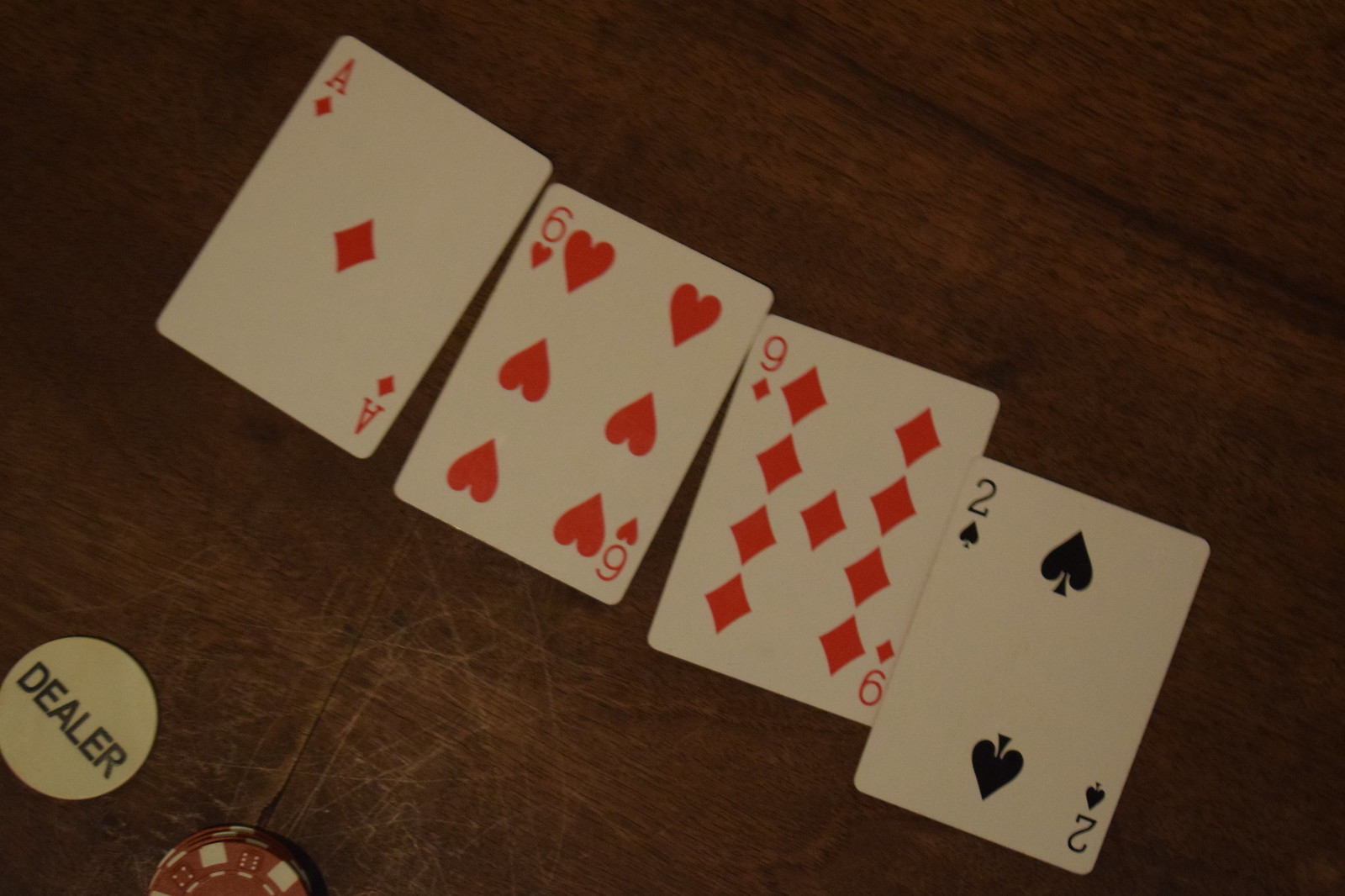An intense poker game scene is captured atop a dark, stained wooden surface, marked with time and a few scratches. At the bottom left, a white dealer chip inscribed with "DEALER" in bold, black Arial font stands out prominently. Adjacent to the dealer chip is a partially visible stack of poker chips, colored red and white, hinting at the competitive atmosphere. Arranged diagonally from the top left to the bottom right, four playing cards lie on the wooden table. The cards, in order, are an ace of diamonds, a six of hearts, a nine of diamonds, and a two of spades. The ace of diamonds, positioned at the top left, stands apart from the rest. Below it, the six of hearts and nine of diamonds slightly overlap at their top corners, creating a cohesive line. The arrangement concludes with the black two of spades, overlapping the very edge of the nine of diamonds, but leaving all the numbers and the diamond symbols unobstructed. This meticulous setup amplifies the drama and anticipation in the midst of a high-stakes game.